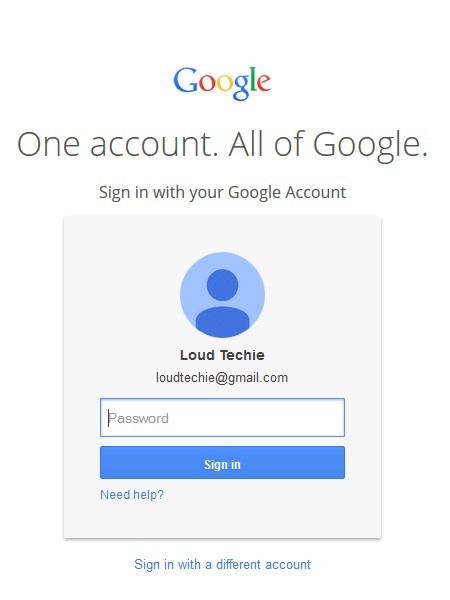This full-color image depicts a Google sign-in screen. The background is predominantly white, creating a clean and minimalist interface. Dominating the top center is the iconic Google logo, featuring its signature colors: blue, red, yellow, green, and another blue and red. Below the logo, the text reads, "One account. All of Google."

Beneath this statement, a prompt encourages users to "Sign in with your Google Account". The main focus of the image is a grey login box. Inside this box, a blue circular avatar, representing a user icon, displays a dark blue circle enclosing a lighter blue circle with simplistic blue shoulders. 

Directly below the avatar, the name "Loud Techie" is displayed, accompanied by the email address "loudtechie@gmail.com." There is an empty password input field ready for the user to type their credentials. The prominent blue "Sign in" button sits below the password field, with "Sign in" inscribed in grey text.

To the bottom left of the sign-in button is a hyperlink in blue text reading, "Need help?" A thin, grey horizontal line separates this segment from the text below it. At the very bottom center of the interface, additional blue text offers the option to "Sign in with a different account.” The overall presentation is a typical Google login interface, clear and functional, guiding the user efficiently through the sign-in process.